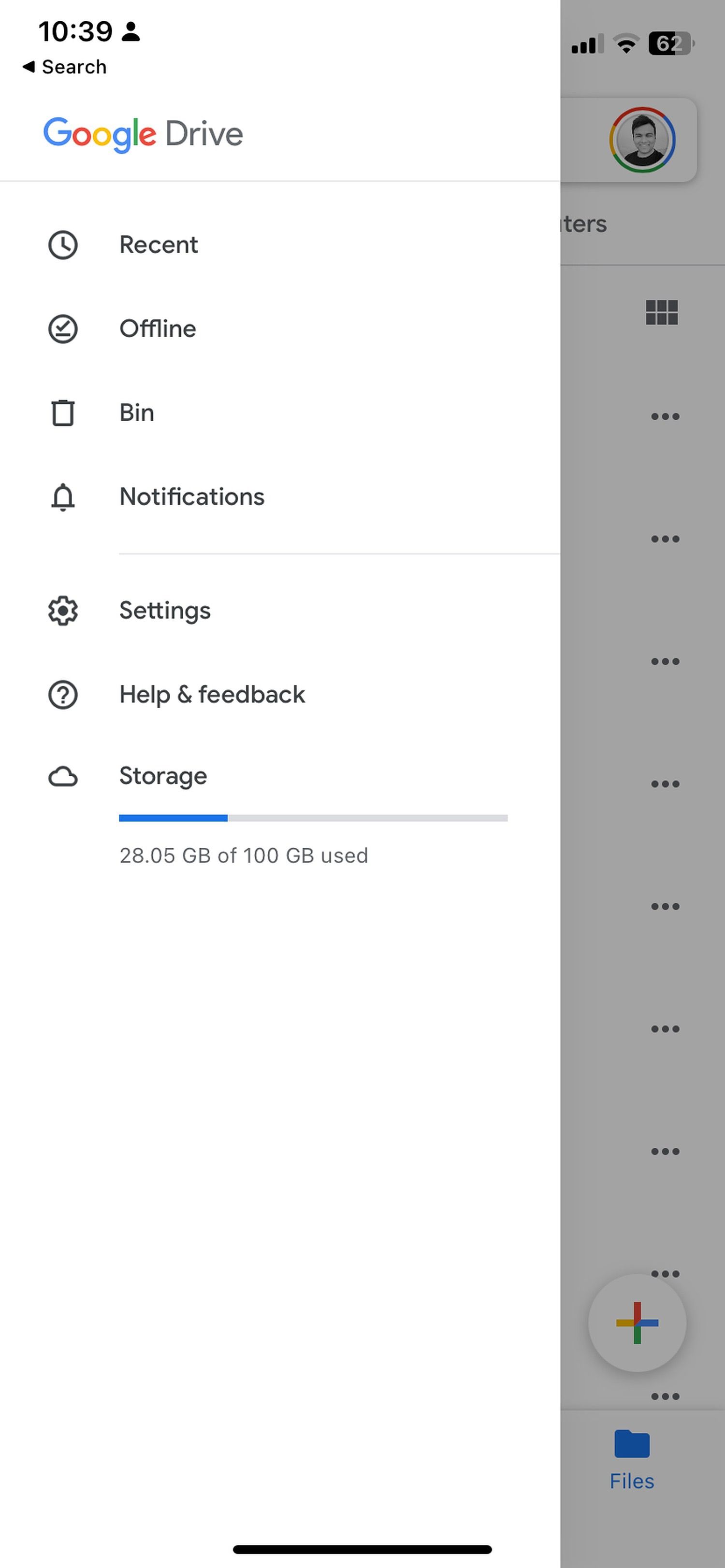Screenshot Description:

A mobile screenshot showcasing the interface of a Google Drive page on an Android device. The screen is divided into two parts: the left side displays an overlay menu while the right side shows a partial view of the main Google Drive interface.

In the overlay menu, the header reads "Google Drive". Below this are several options, each accompanied by an icon:
- **Recent:** A clock icon.
- **Offline:** An icon of a checkmark with a line underneath it encased in a circle.
- **Bin:** A trash can icon.
- **Notifications:** A bell icon.
- **Settings:** A cogwheel icon.
- **Help and Feedback:** A question mark icon.
- **Storage:** A cloud icon. Next to it, the storage usage is displayed as "28.05GB of 100GB used".

The background of the overlay menu is predominantly white. To the right, we can glimpse the main Google Drive layout, with multiple file listings each featuring three vertical dots for additional options.

In the top right corner of the screenshot, there's a small, black-and-white profile image of a person, which is too small to discern clear details. The time displayed at the top left corner is "10:39".

At the bottom right, there's a blue folder icon labeled "Files". Above it, there's a white circle with a multicolored plus symbol, likely for adding new files or folders.